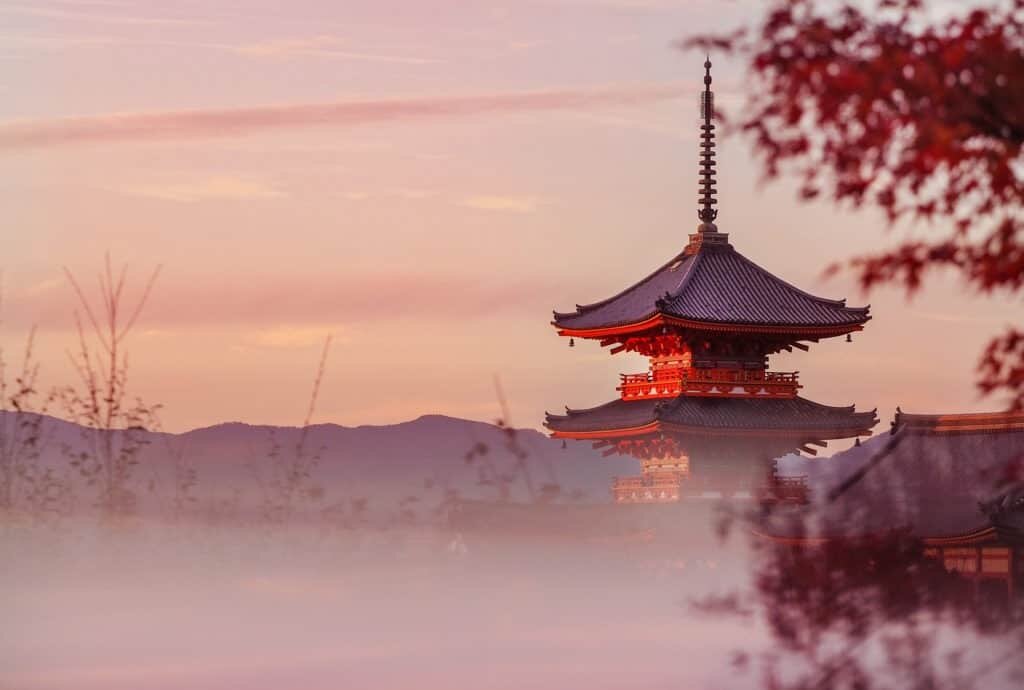This color photograph captures a serene Japanese landscape featuring a traditional pagoda set against a backdrop of bluish-gray sky and narrow clouds. The pagoda, characterized by its distinctive red wood and ornate design, stands prominently with two levels of gray roofs. Perched atop the structure is a dark gray metal spire extending into the sky. 

In the distance, blue mountain tops rise gently, adding to the tranquil atmosphere. The foreground is dominated by blurred red leaves from a nearby tree, suggesting depth and enhancing the focus on the pagoda. Below the pagoda, the ground is veiled by a layer of mist, partially obscuring details yet revealing patches of grass and small shrubs above the haze. The hazy effect gives an impression of elevation or atmospheric conditions like precipitation. 

Additionally, another structure with a gray roof is faintly visible to the near right, though details are obscured. Overall, the image melds architectural elegance with natural beauty, creating a captivating and tranquil scene.